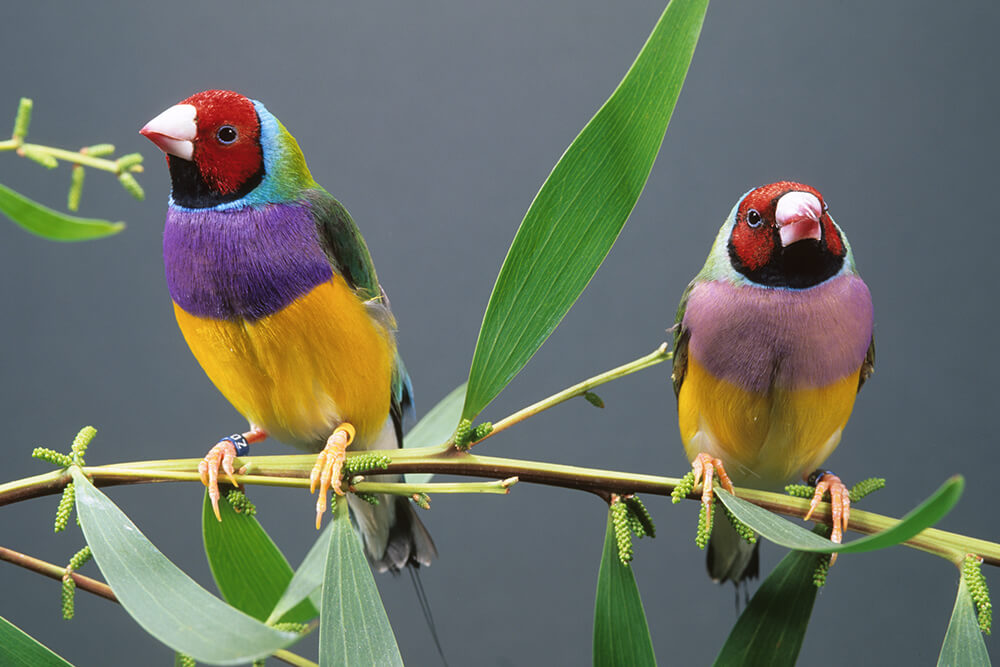In this vibrantly detailed, color photograph in landscape orientation, two brightly colored parakeets perch on a thin tree limb against a deep blue background. The birds are positioned at opposite ends of the branch, with the left bird facing left and the right one facing forward, a lush leaf rising between them. Both birds exhibit similar striking markings. The bird on the left has a bright purple chest, yellow abdomen, green wings, and a blue band on its leg. Its beak is white tipped with red, and under its black lower beak, a vivid red spreads across the cheeks and over the head, transitioning to a light blue strip and various shades of green at the back. The bird on the right, with a slightly lighter purple chest, mirrors these hues with a light blue neck ring, green wings, yellow belly, and similar banded leg and beak details. Photographic realism captures the dynamic interplay of forest green, light purplish pink, and other vivid colors, accentuating the lively essence of these charming creatures.